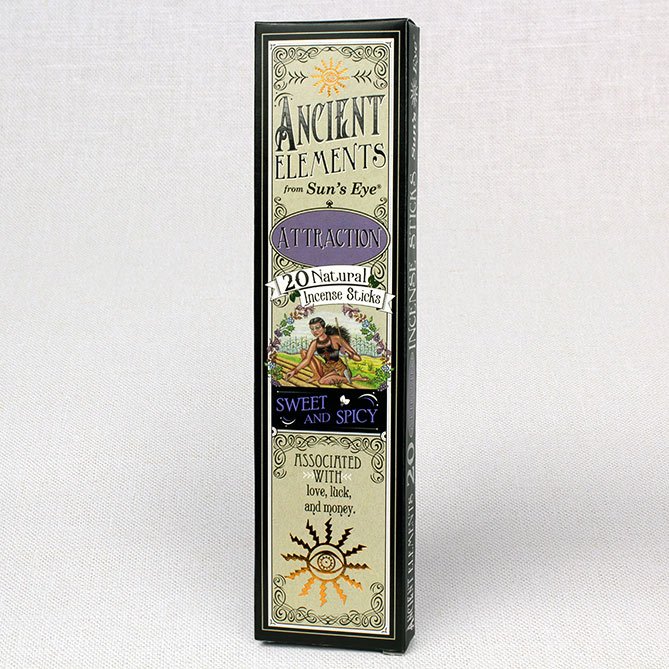The image depicts a black rectangular box standing upright against a gray background. The box features a detailed label with multiple elements and text. At the top, there's a yellow sun adorned with intricate designs, followed by the text "Ancient Elements from Sun's Eye" in black lettering. Below, an oval with a purplish-blue color contains the word "Attraction" in black text. Directly beneath this, two white banners display "20 Natural Incense Sticks" in black writing. The central part of the label showcases a drawing of a Native American woman with long black hair, wearing a tank top and brown skirt, kneeling in a green field dotted with flowers with green leaves and purple petals. Another banner below reads "Sweet and Spicy" in blue text. At the bottom, an eye symbol surrounded by zigzag lines and lightning bolts emphasizes themes of love, luck, and money, stating "Associated with Love, Luck, and Money." Overall, the box is a package of incense sticks that combines artistic imagery with text, suggesting it brings positive attributes through its use.